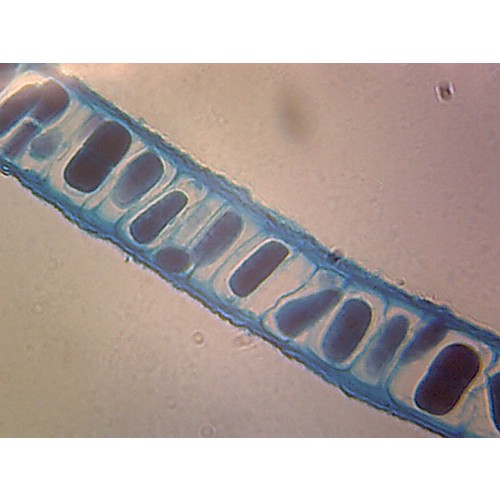The image depicts a detailed microscopic view of cells arranged diagonally from the upper left-hand corner to the lower right-hand corner. The background transitions from a pink-peach color on the right side to a pale green-gray on the left, with hints of tan and purple, indicating different zones of focus and lighting under the microscope. The central focus is a group of 12 cells, each surrounded by distinct, wavy blue lines and thin light-blue membranes. The cells themselves appear dark grayish-brown and are structured with separations, giving them a bean or capsule-like appearance. Some lighter areas and blurred silhouettes of additional cells, along with scattered bubbles, can be seen in the background, adding depth to the close-up image. This highly magnified view highlights the intricate cell walls and inner segments, making it a fascinating study of cellular structure.